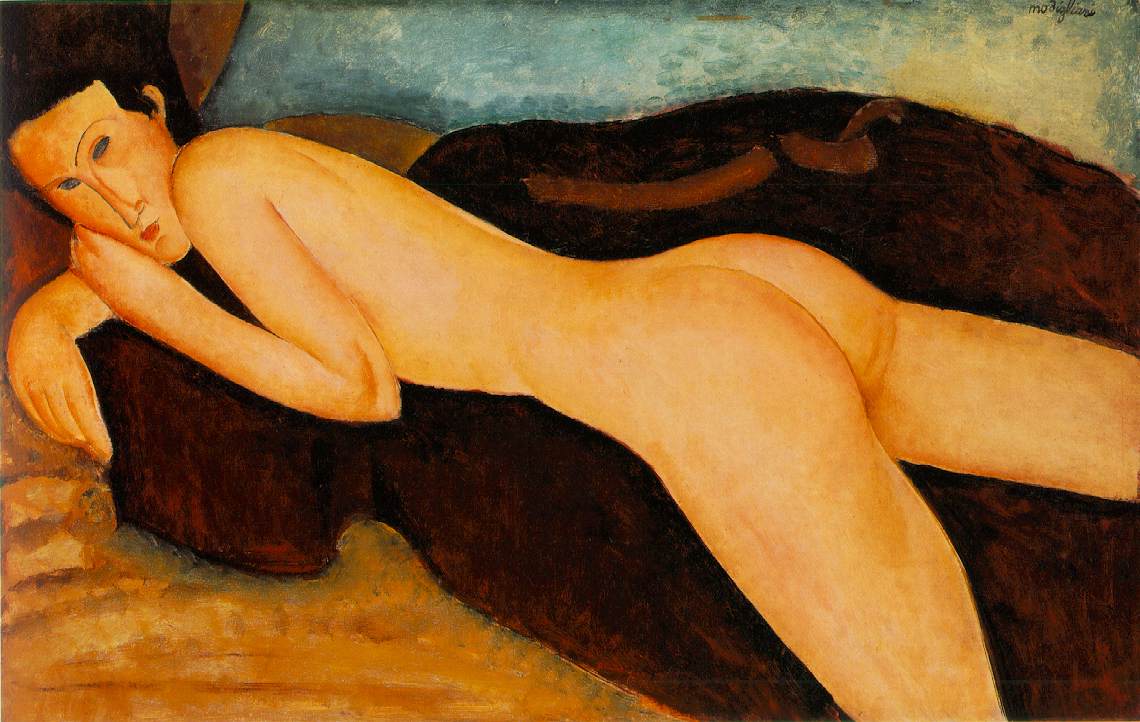An oil-based painting with both slightly realistic and angular, two-dimensional style portrays a nude individual lying on their stomach on a large, brown object resembling a couch or table. This figure, with a smooth, curvaceous form, short dark hair, and skin painted in yellowish-orange hues, has their back and bottom facing upward. Their left elbow is bent, propping their chin with their left hand, while their right arm lies beneath them. The face features minimalistic details with narrow, slanted eyes, a long nose, and tiny red lips. Surrounding the figure is a background of mustard beige and brownish-orange tones, complemented by splotches of blue and a hint of a yellow sun. In the top right corner, a signature is visible against the light blue expanse reminiscent of a sky.